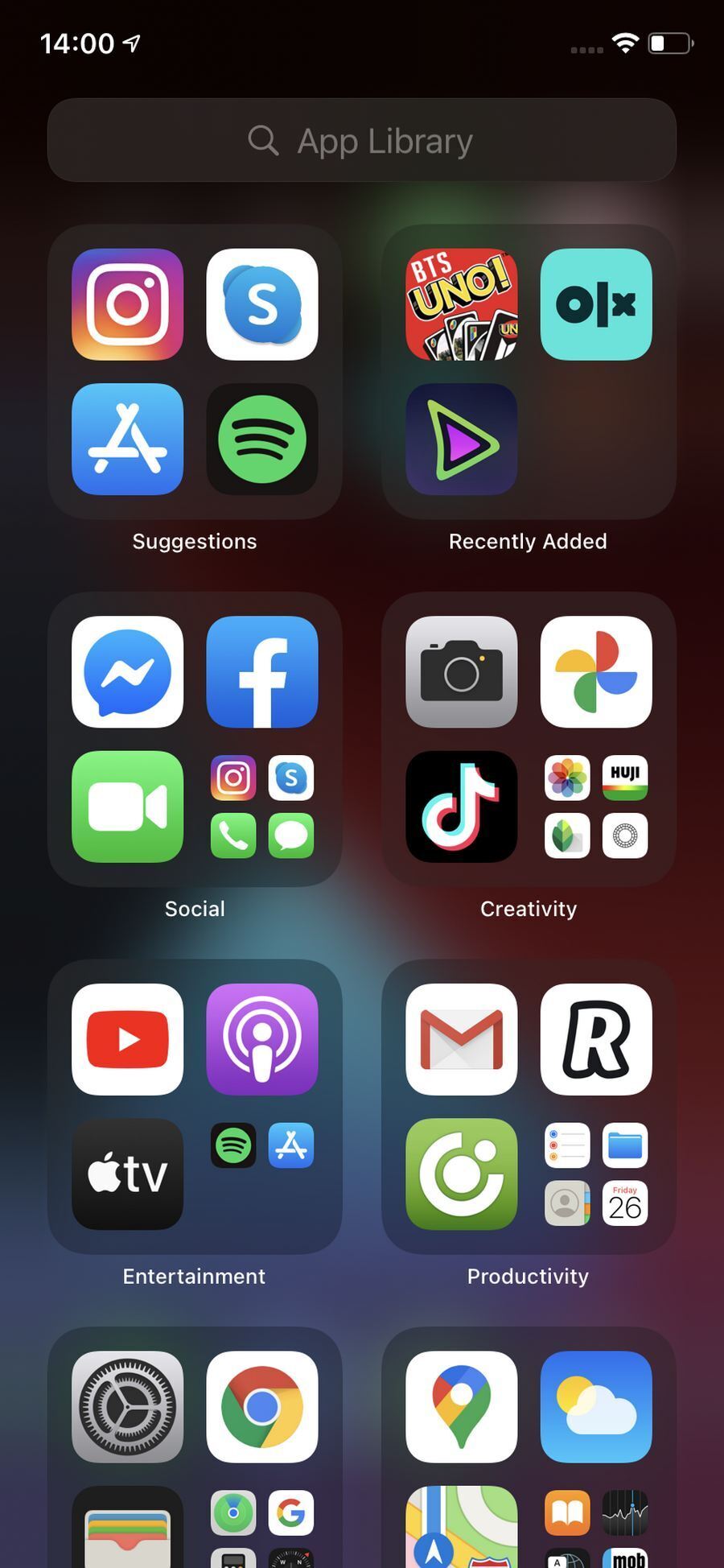The image showcases a screen under the header "App Library," displaying a variety of apps systematically grouped into categorized squares. There are eight primary grouped sections arranged in a 2x2 grid with an additional row partially visible at the bottom. Each of these squares contains a collection of app icons, organized under relevant categories.

The categories from left to right are as follows: "Suggestions," "Recently Added," "Social," "Creativity," "Entertainment," and "Productivity." The further categories at the very bottom are obscured from full view. Specifically focusing on the "Social" category, within it are app icons for Messages, Facebook, and a video-related app. There is also a smaller nested square within the "Social" category, containing Camera, Phone, Messages, and an icon labeled with a '5'.